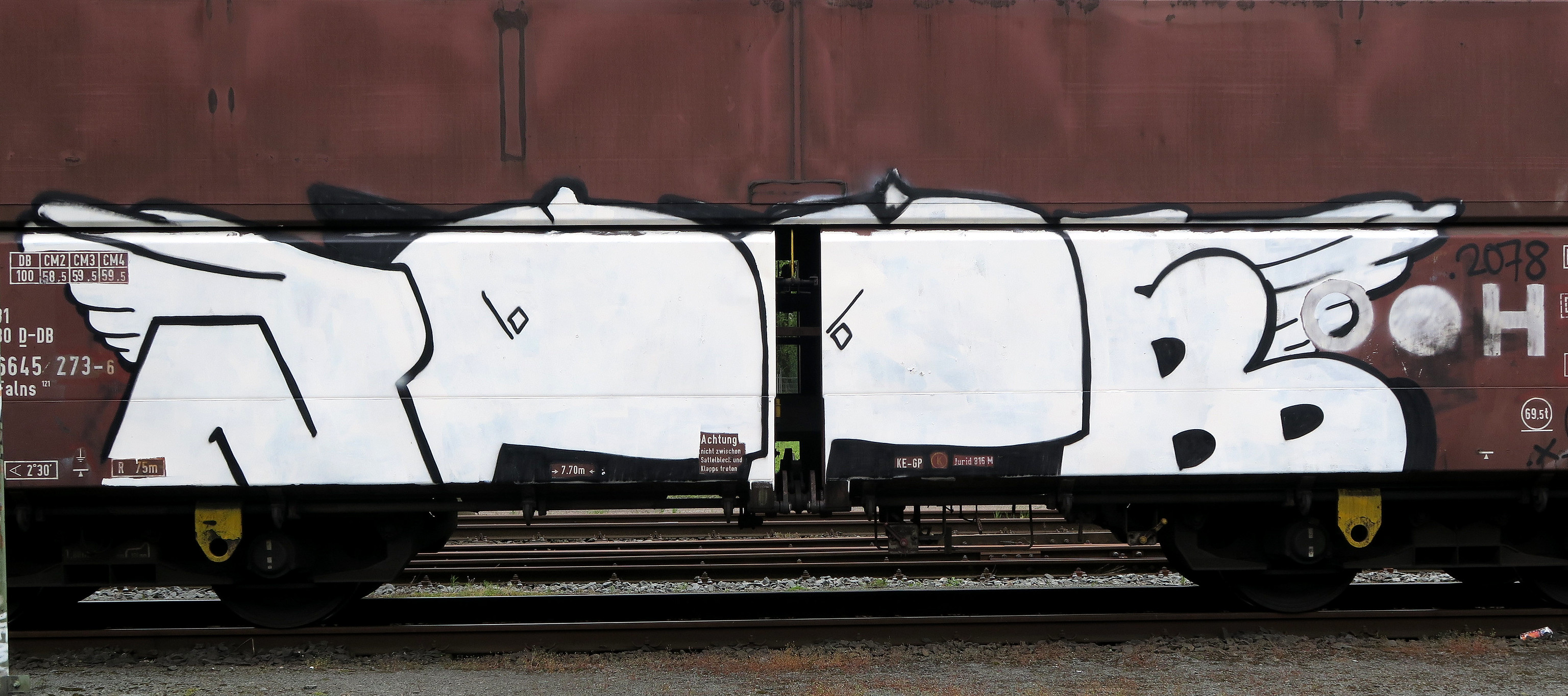This photograph depicts the lower portion of a train car painted in a dark rust red or maroon color, with the top of the car not visible in the image. The train car, set against a gravel or dirt surface with visible train tracks, features intricate graffiti artwork occupying the bottom half. This vibrant white graffiti is outlined in black and includes a mix of illegible lettering and distinctive designs. The left and right ends of the graffiti each feature symmetrical wing motifs, with the right wing resembling a 'B' shape. In the middle, there are two symbols: one with a line on the left and a diamond on the right, and another with a line on top and a diamond on the bottom, which some interpretations suggest resemble creatures or possibly whales with wings. The train car's undercarriage shows two connected sets of wheels, and there is a small yellow metal piece hanging off. Some partial white numbering is present on the left edge of the car, though it's cut off and unreadable. Overall, the graffiti appears freshly painted, contrasting vividly with the aged, rusty surface of the train car.